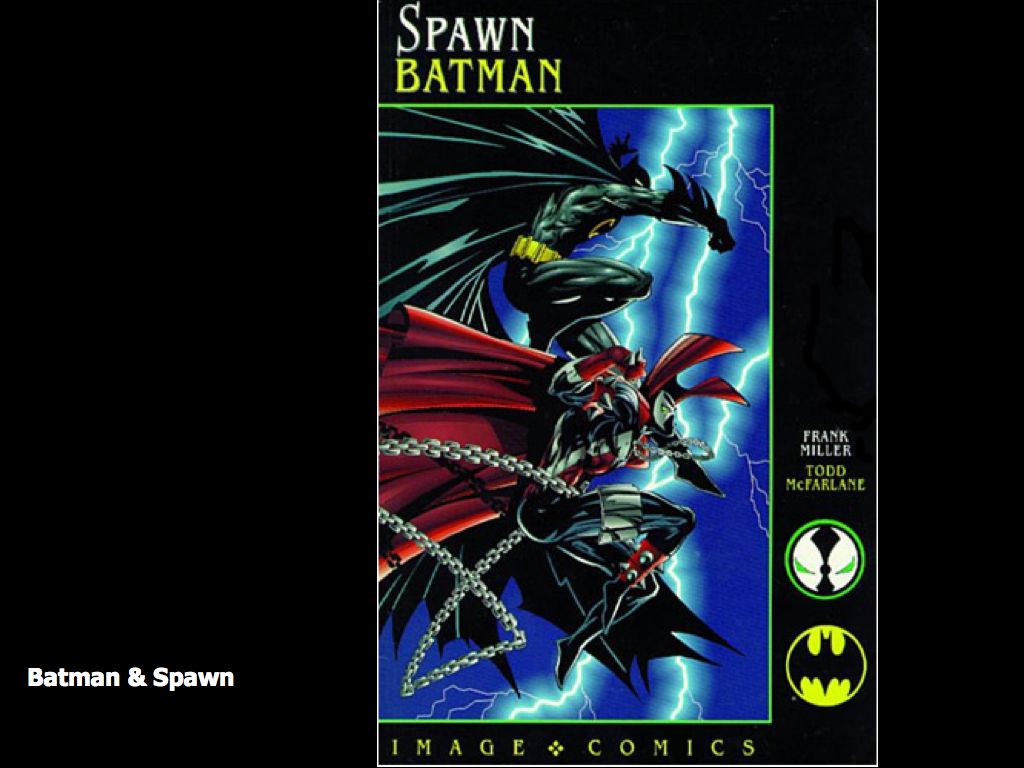The image is a detailed front cover of a classic comic magazine titled "Batman Spawn" by Frank Miller and Todd McFarlane, likely from the 70s or 80s. The cover features a dynamic cartoon artwork depicting Batman in a crouched position with his cape flowing dramatically behind him. Batman is positioned above another character who is identified as Spawn. Spawn is adorned in a red vest with metal chains, black shiny pants, and red spikes on his legs, giving him a villainous appearance. The scene is set against a background lit by a lightning bolt, enhancing the dramatic effect. The cover is framed with a green border. On the top left, the titles "Spawn" and "Batman" are displayed in white and yellow text respectively. The bottom right corner features the iconic Batman logo with its yellow and black color scheme, along with another symbol resembling a green-eyed figure. The names "Frank Miller," "Todd McFarlane," along with the words "Image Comics" are prominently displayed at the bottom of the cover.